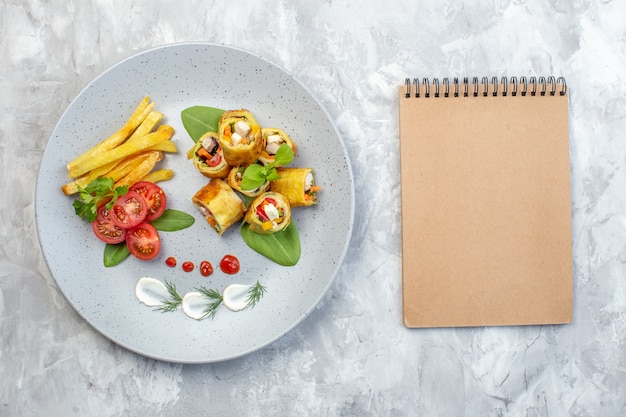The image showcases a visually appealing arrangement of food and a notebook on a clean, marble-like, concrete surface. Central to the scene is a white plate positioned slightly to the left. The plate features an eclectic mix of culinary items: on the left side, a few french fries and sliced tomatoes rest atop a small bed of greenery; on the right, a collection of open-ended pastry rolls, resembling taquitos or tater tots, are filled with cheese, corn, and diced tomatoes, and accompanied by some leafy greens underneath. At the bottom edge of the plate are three dollops of white sauce, each topped with a sprig of greenery. Adjacent to the plate on the right-side sits a brown notebook, face down, adding a casual yet stylish element to the setting. The overall color palette of the image includes shades of brown, green, red, white, gray, and tan, creating an inviting and appetizing visual display.